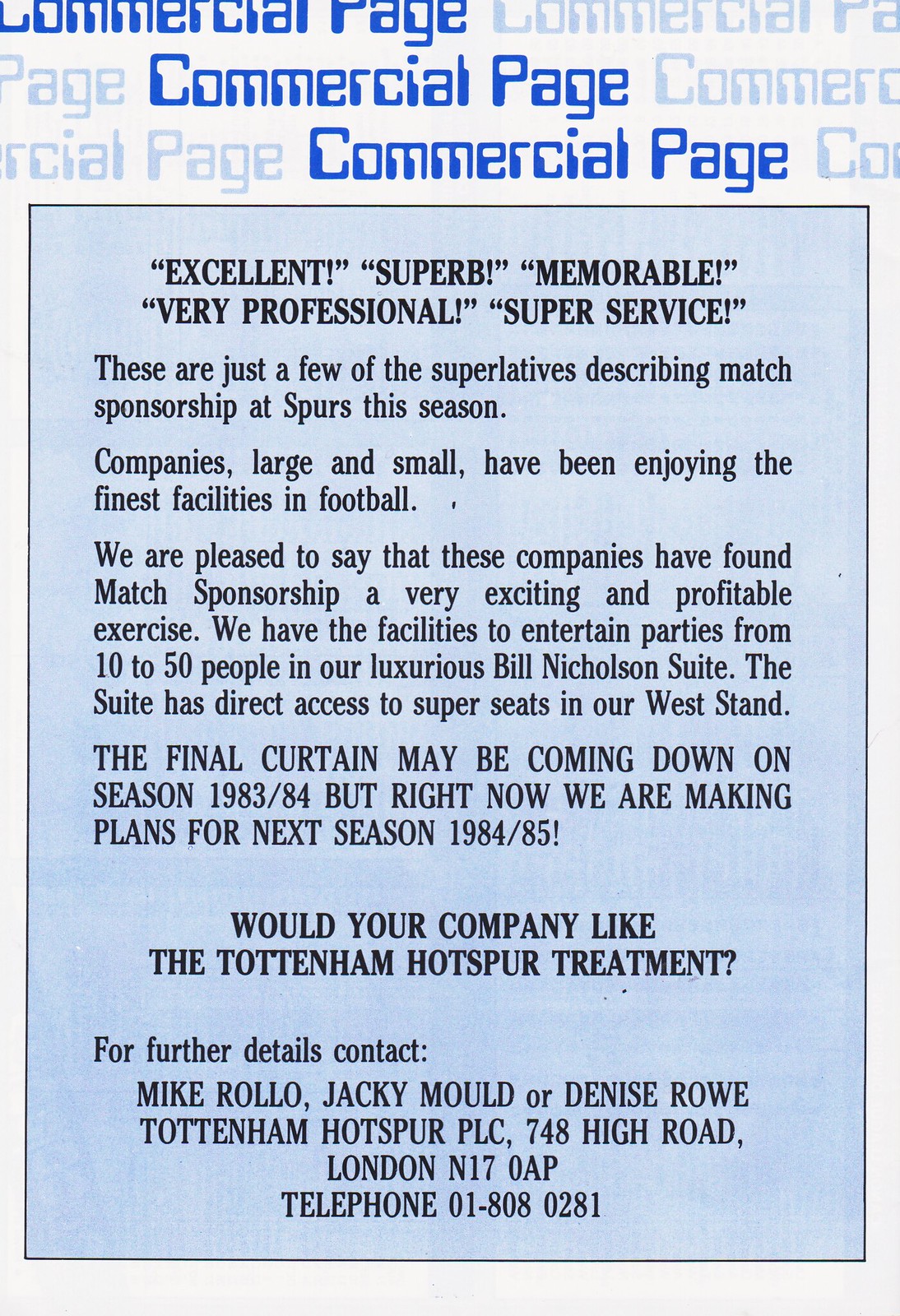The image displays a tall rectangular advertisement with a light gray background. At the top, in alternating dark blue and light blue fonts, the phrase "commercial page" is repeated multiple times. Just below, a prominent light blue rectangle with a thin black frame contains the text: "excellent, superb, memorable, very professional, super service." This section describes the exceptional qualities of match sponsorship at Spurs. The advertisement highlights that companies, both large and small, have enjoyed the exceptional facilities, noting that match sponsorship has proven to be an exciting and profitable venture. Specifically, it mentions the luxurious Bill Nicholson suite, which can accommodate parties of 10 to 50 people and provides direct access to prime seats in the West Stand. Although the 1983/84 season is ending, plans are already underway for the 1984/85 season. The ad, in all caps, asks if companies would like the "Tottenham Hotspur treatment," providing contact details for further information: Mike Rolo, Jackie Mould, or Denise Rao at Tottenham Hotspur PLC, 748 High Road, London, N17 OAP, telephone 01-808-0281.